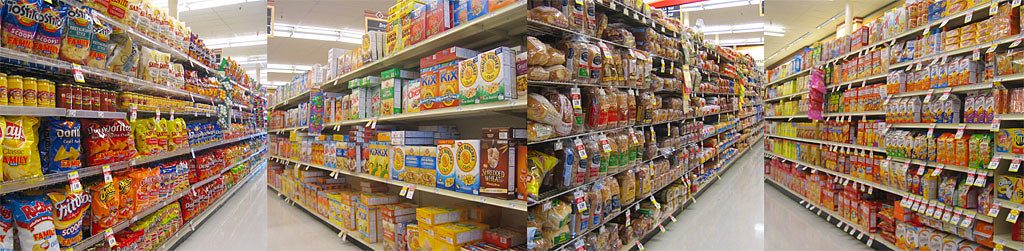This image is a composite of four photographs each depicting different aisles inside a grocery store. The first photo, located on the far left, shows a vibrant snack aisle lined with various kinds of chips and dips. Visible brands include Tostitos, Lay's, Doritos, Ruffles, Fritos, and Cheetos, all displaying a spectrum of colors—blue, yellow, red, orange, and green. Alongside the chips, there are bottles of cheese dip and salsa, arranged on different shelves. The next photo showcases an aisle dedicated to cereals. Clearly identifiable are boxes of Kix, Honey Bunches of Oats (both with and without almonds), Chex, and Golden Grahams, featuring a lively mix of colors like red, blue, green, yellow, orange, and brown. The third image shifts focus to the bread aisle. Although specific brands are not discernible, various types of bread such as rye, pumpernickel, white, and Italian loaves are visible, stacked in colorful packaging—red, green, blue, and white. The red, white, and yellow tags hanging from the shelves suggest sales and special deals. The final photograph to the far right highlights a row filled with assorted snack crackers. Prominently featured are Goldfish crackers and various kinds of Ritz, accompanied by cookies and Cheez-Its. This aisle, too, bursts with a vivid array of colors—purple, orange, yellow, green, blue, red, and white. Each photograph also reveals the store's bright, fluorescent light fixtures on the ceiling and a shiny tile or linoleum floor, enhancing the overall clarity and brightness of the scene.